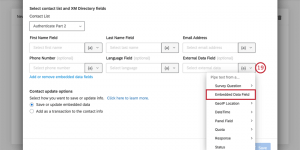Screenshot of a Form Interface on a Dark Gray Background

This image is a screenshot of an unidentified software interface presented on a dark gray background. The prominent textual elements are mostly illegible due to significant blurriness. However, a few sections can be discerned, including labeled fields such as "Contact List," "Find Name Field," "First Name Field," "Last Name Field," "Email Address," "Phone Number," and "Language Field." There is a dropdown menu, also too blurry to read, positioned near a highlighted area outlined in red. Additionally, there is a red circular icon with the number "19" prominently displayed within it, located above and to the right of the outlined area. The image is rectangular, wider than it is tall, and lacks any photographic elements or depictions of people, animals, plants, buildings, vehicles, or airplanes. Overall, the screenshot appears to be of a user interface form, but the majority of its content remains indistinct due to the poor clarity of the image.